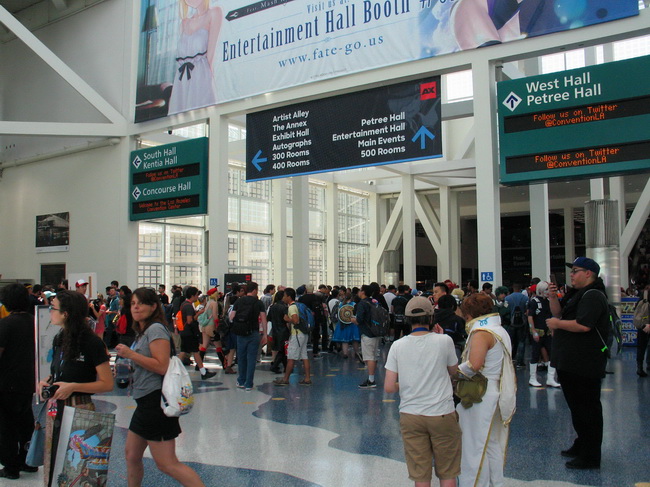The image is taken indoors, resembling the bustling environment of an exhibit or convention hall. In the foreground, several people are milling about, walking in different directions, contributing to a lively and somewhat chaotic atmosphere. The large, open space features several steel support columns and expansive glass windows situated toward the left, allowing natural light to flood in. The blue tiled floor, accented with an irregular pattern of white tiles, further defines the expansive area. 

A prominent banner hangs across the top, partially cut off, reading "Entertainment Hall Booth, www.fate-go.us". Below this, additional signage directs attendees to various locations within the hall, including "Artist's Alley, the Annex, Exhibit Hall, Autographs, 300 rooms, 400 rooms" with an arrow pointing left. Other signs provide further guidance, indicating areas such as "West Hall, Petrie Hall, South Hall, Kinesia Hall, Concourse Hall" and more, highlighting both destinations and accessibility features. In the background stands a blue and yellow booth, likely part of the exhibition setup. The structure of the building, with its white-painted interior and steel posts, gives it a polished, industrial look, suitable for hosting major events.

In summary, this detailed interior view captures the dynamic and organized chaos typical of a major convention hall or exhibition space, complete with a diverse crowd, clear directional signage, and a robust architectural framework.